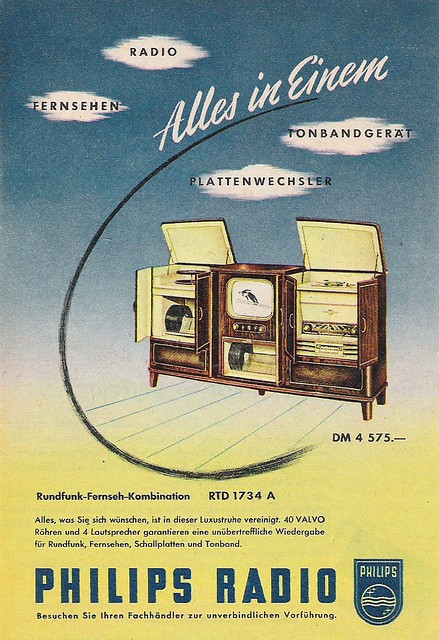This image is a detailed poster showcasing an advertisement for an old Philips radio console, likely from the 1950s or 60s. The poster features a drawing of a large, ornate wooden cabinet that opens up to reveal a central screen resembling an old television, flanked by various compartments. The left compartment appears to house a record player, and below the central screen, there's space allocated for storing records. The text on the poster includes German words such as "Alles in Einem," "Fernseher," "Platten," "Wechsler," and "Tonbandgerät," indicating it’s a multi-functional entertainment unit. At the very bottom of the poster, the text "Philips radio" is prominently displayed in blue. The background of the poster transitions from a dark blue at the top to a yellow hue at the bottom. The model number "D-M-4575" is also mentioned, emphasizing its specific model designation. Overall, the advertisement highlights the sophisticated design and multifunctionality of the Philips radio console.